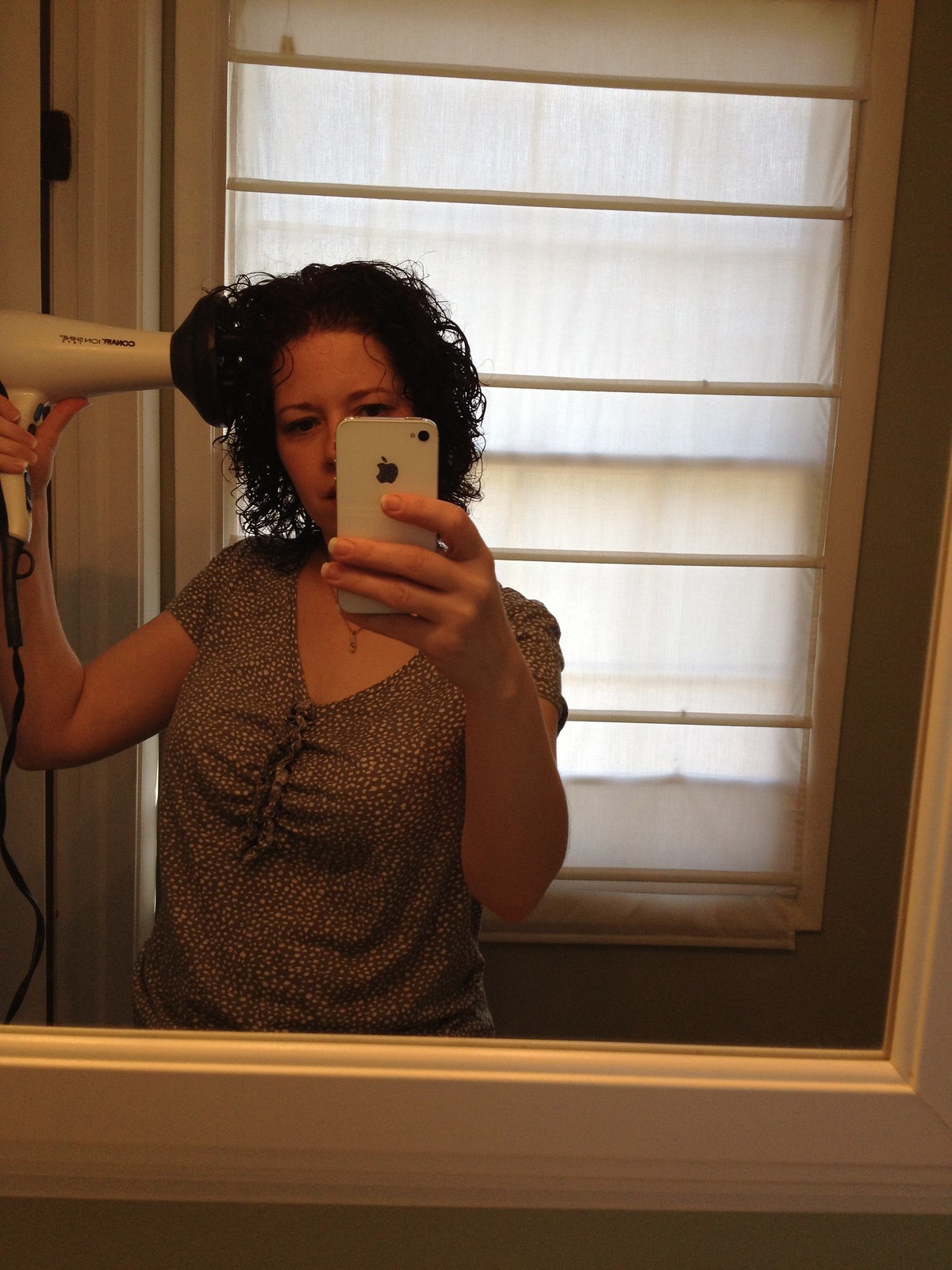In this detailed portrait-style photograph, a Caucasian woman with wet, black, shoulder-length curly hair is taking a mirror selfie. She holds a white iPhone with a single camera in her left hand, which partially obscures three-quarters of her face. In her right hand, she holds a white hairdryer equipped with a wider black nozzle designed for curly hair, its cable extending downward. The woman, who is dressed in a short-sleeved brown blouse adorned with white dots, stands in a small room. The mirror's white-painted wooden frame features intricate moldings and crevices, reflecting a window behind her covered by translucent white Roman or Holland blinds, allowing diffused light to filter through. The room's visible walls show a contrast, with the wall behind her appearing darker. Additionally, a doorway extends outward from the left side of the image, contributing to the intimate setting of the scene. The woman's curious expression adds a touch of personality to this meticulously captured moment.